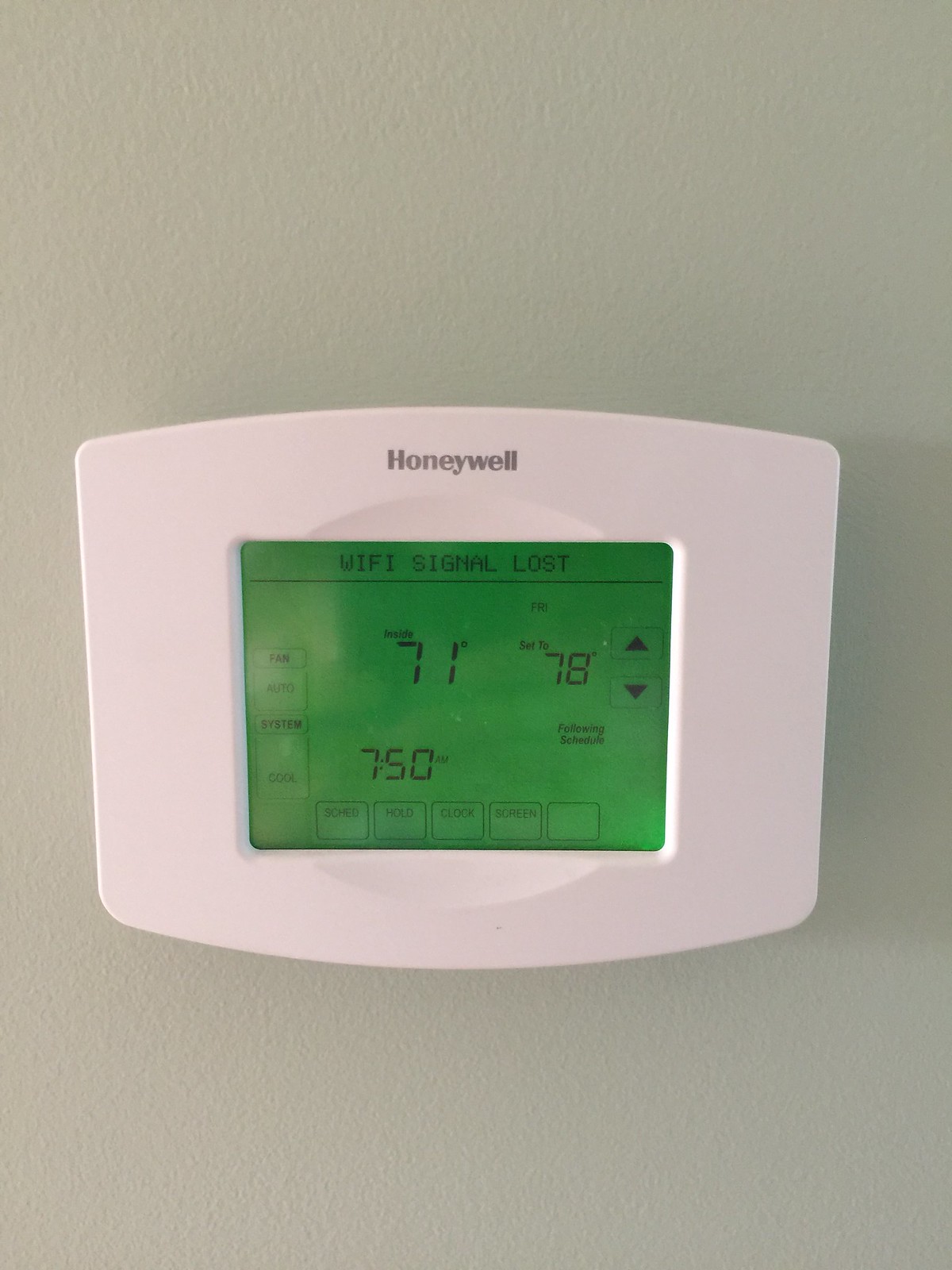A high-resolution photograph of a wall-mounted Honeywell thermostat is depicted. It is affixed to an off-white, slightly greyish painted sheetrock wall with a subtle orange peel texture. The thermostat itself is a white plastic rectangular device, featuring an illuminated digital display. The screen has a green backlight with black text and numbers. It shows a message "Wi-Fi signal lost" and displays the current temperature of 71°F. On the far-right side of the display, "78" is shown next to up and down arrows, likely indicating setpoint adjustment controls. The time at the bottom of the screen reads 7:50, although it is unclear whether it is a.m. or p.m.

Surrounding the edges of the display are several small squares that appear to be touch-sensitive controls. These include options labeled "Fan," "Auto," "System," "Cool," and along the bottom, partially readable labels for what seem to be "Schedule," "Hold," "Clock," "Screen," and an unlabeled button. The photograph appears to be taken under natural lighting, casting a faint shadow to the right of the thermostat, suggesting the light source is coming from the left side of the image.